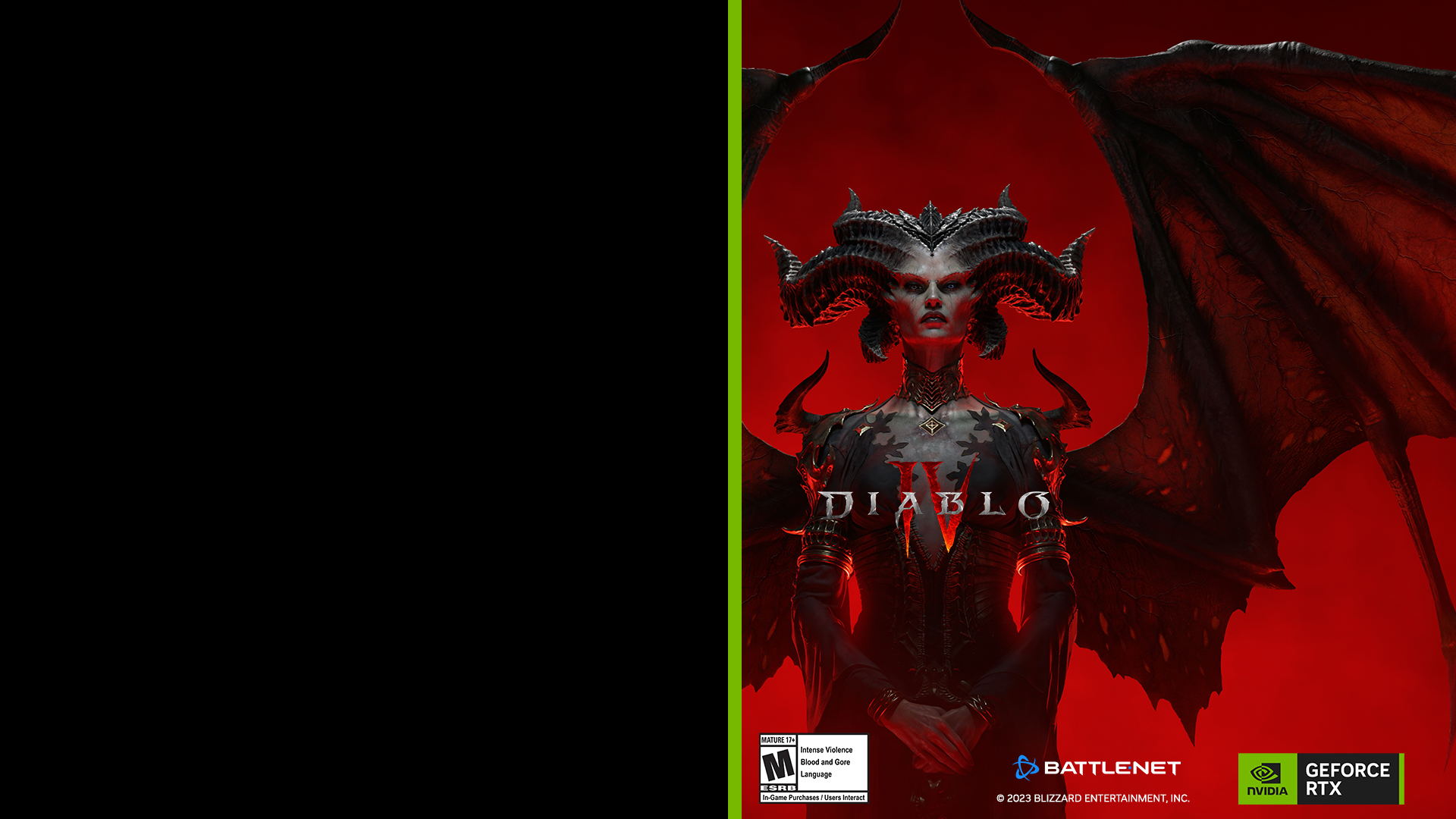This image is divided into two halves. The left half is a solid black square with a vertical lime strip running top to bottom at the center, separating it from the right half. The right half is the cover of the video game "Diablo IV" set against a deep red background. Dominating the cover is a fearsome mythical creature resembling Medusa, dressed in a long black outfit with a high collar. Her face is adorned with serpentine-like appendages that extend backward from where her ears should be. Large, imposing black wings rise from her lower back to the top right corner of the image, though the wing on the left is partially cut off. In bold white letters, the title "Diablo" is displayed across her chest, with the Roman numeral IV (4) in red beneath it, signifying "Diablo IV." Below this, the white Battle.net logo appears, followed by the text "2023 Blizzard Entertainment Inc." in smaller print. At the bottom left corner of this panel, a white sticker indicates a mature audience rating due to increased violence, blood, and gore. To the right of the Battle.net text, there's another rectangular section with a black background featuring the 'GeForce RTX' logo, next to the green Nvidia logo.